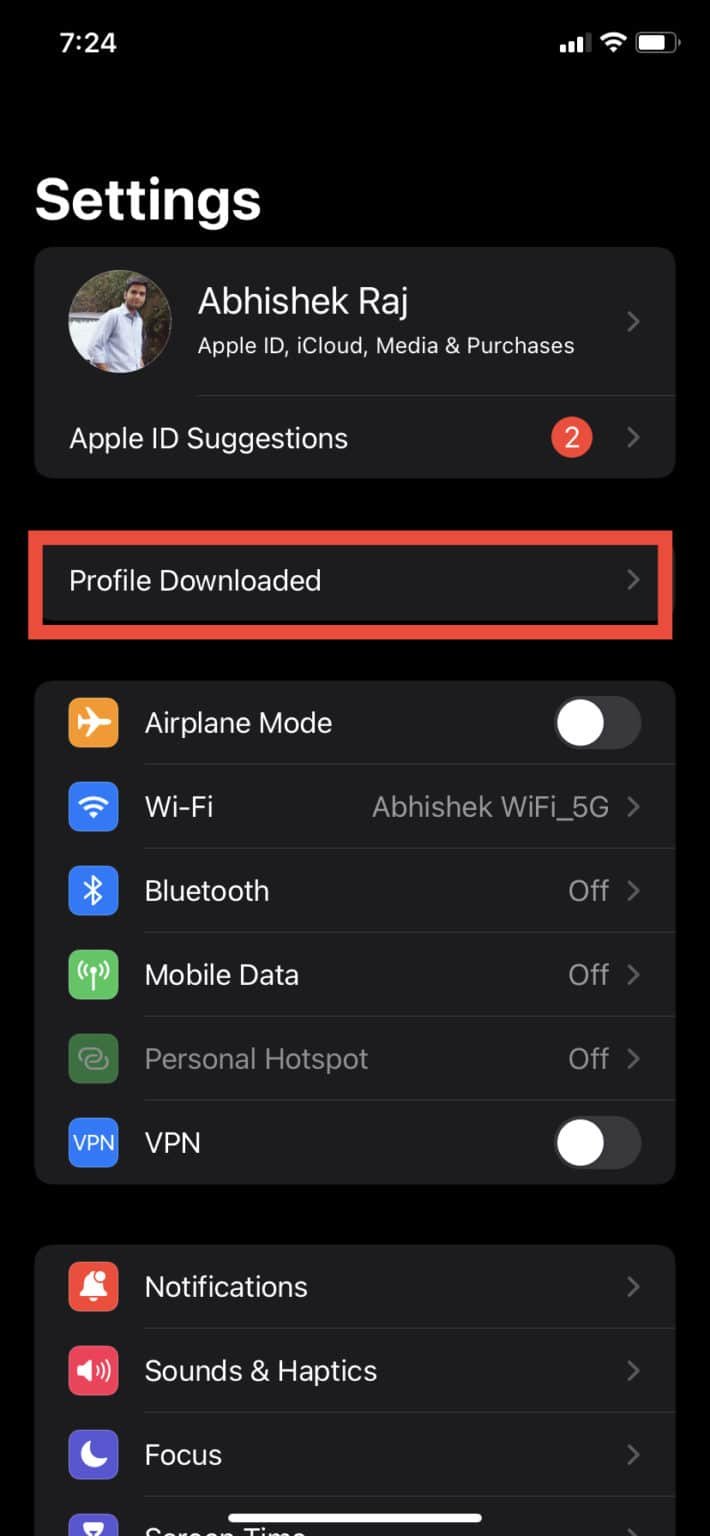The screenshot displays a cell phone screen in dark mode. At the top of the screen, the time is shown as 7:24. In the upper right corner, icons indicate a battery level at about 90% charged, a full Wi-Fi signal, and 3 out of 4 bars from the cell phone tower. Below the time, the word "Settings" appears in white letters. 

Directly underneath this, there is a rectangular section displaying the user's profile information: "Abkhyshek Raj, Apple ID, iCloud, Media & Purchases," accompanied by a right-pointing arrow and the user's profile picture in a circular frame. Below this, "Apple ID Suggestions" is displayed alongside a red circle with the number 2 inside it, and another right-pointing arrow.

Further down, there is a red rectangle labeled "Profile Downloaded," also with a right-pointing arrow inside the red rectangle. 

Continuing downwards, the list of settings includes:
- "Airplane Mode" with the toggle switch set to off.
- "Wi-Fi," showing "Abkhyshek Wi-Fi 5G" with a right-pointing arrow.
- "Bluetooth," which is off, with a right-pointing arrow.
- "Mobile Data," which is off, with a right-pointing arrow.
- "Personal Hotspot," which is off and ghosted out, with a right-pointing arrow.
- "VPN" with the toggle switch set to off.
- "Notifications" with a right-pointing arrow.
- "Sound & Haptics" with a right-pointing arrow.
- "Focus" with a right-pointing arrow.